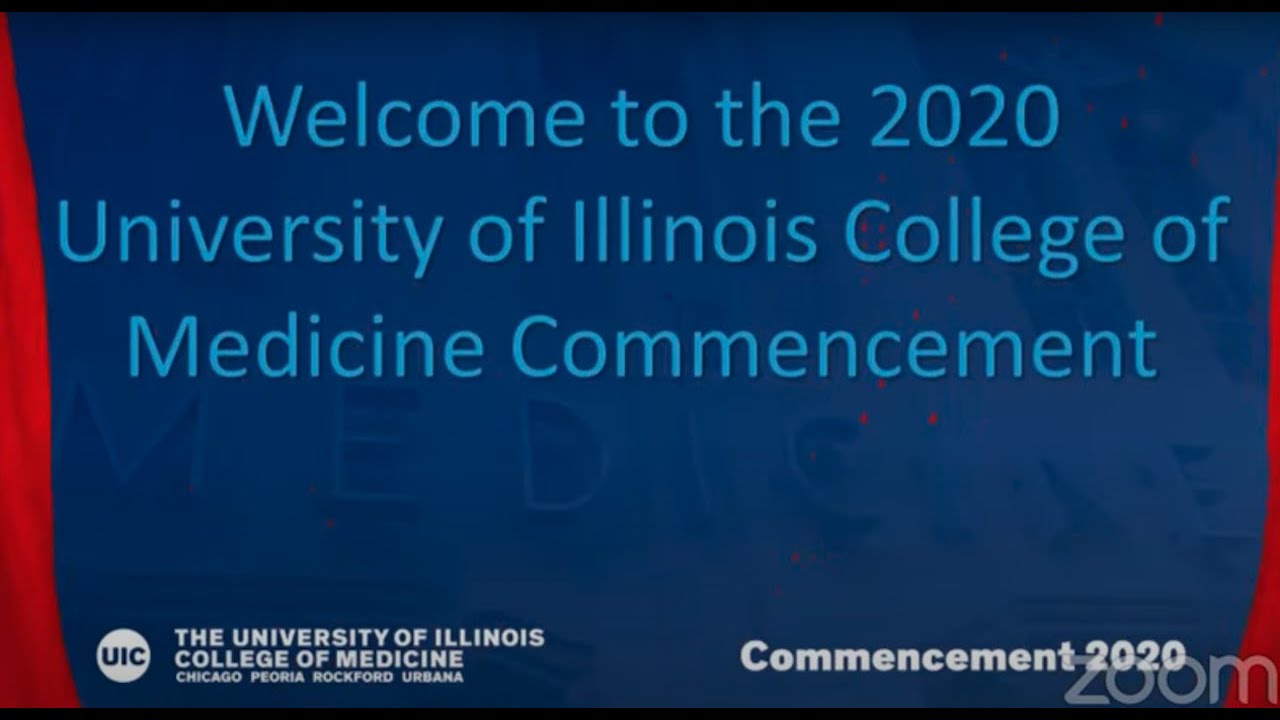The image features a rectangular design with a sophisticated blend of navy blue and red hues. The navy blue background serves as the primary canvas, overlaid with striking graphical elements. On the left side, a thin red line cascades down, gradually thickening to mimic the appearance of flowing fabric. This motif repeats on the right side, starting about a fifth of the way down, where a thin red line similarly expands into a broader, fabric-like flow.

In the center, the text "Welcome to the 2020 University of Illinois College of Medicine Commencement" is prominently displayed in a lighter shade of blue, standing out clearly against the dark background. To the right, a white icon representing the University of Illinois College is positioned at approximately the same height.

Below the icon, in white text, the university’s name and campuses are listed: "University of Illinois College of Medicine Chicago Peoria Rockford Urbana." Further to the right, the word "Commencement" is written in capitalized "C" followed by lowercase letters, with "2020" placed immediately beside it.

Subtly intersecting the navy blue and red areas, the word "ZOOM" is inscribed in faint, yet all-uppercase letters, indicating the platform used for the virtual event. The thoughtful layout and detailed elements convey a formal and collegiate atmosphere befitting the commencement celebration.